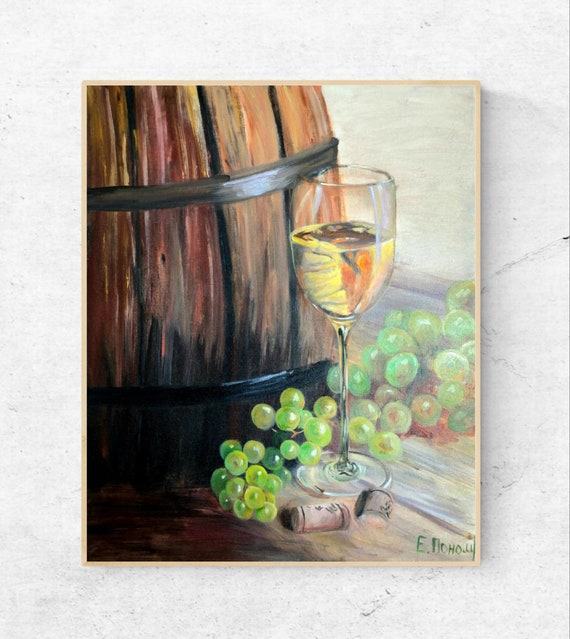The image features a detailed painting of a brown wooden wine barrel adorned with two prominent dark gray ring bands. The barrel is surrounded by an array of green grapes, some tinged with a brownish, reddish hue, and sits atop a surface made of wooden planks with a grayish-creamish brown color. Positioned next to the grapes is a half-full wine glass containing a yellowish, translucent white wine. Two wine corks are visible near the glass. The scene is bordered by a thin wooden frame and rests on what seems to be a marble or marble-like surface. In the bottom right corner of the painting, the artist's initials, "E. H-O-H-O-L-L," are subtly inscribed.